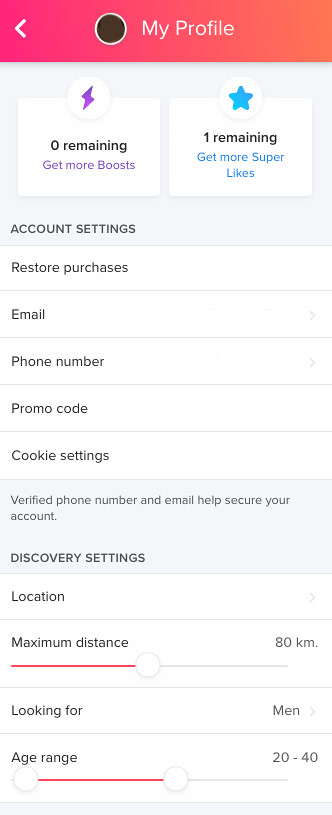Here is a cleaned-up and detailed description of the image:

---

This image is a screenshot taken from a phone, capturing a profile settings page. At the top, there is a prominent banner with a gradient background that transitions from a darker pink on the left to a lighter pink on the right. On this banner, a white left-facing arrow is situated on the far left, followed by a black circle with a white outline, presumably symbolizing an information or profile icon. Next to it are the words "This is my profile," written in white text.

Below this banner, there are two rectangular boxes. The first box reads "0 remaining" and "Get more boosts," accompanied by an icon of a purple lightning bolt within a white circle. The second box states "1 remaining" and "Get more super likes," featuring a star within a white circle.

Further down on the left side, there is the text "Account Settings," which is followed by a dividing line that separates it from the next section. This section includes options such as "Restore Purchases," "Email," "Phone Number," "Promo Code," and "Cookie Settings." Both the "Email" and "Phone Number" sections have right-facing arrows at the end.

At the bottom of the screenshot, there is a gray rectangle containing the text "Verify phone number and email to help secure your account" and "Discovery Settings." Below this, the options include "Location," "Maximum Distance," which displays a slider going up to "80 km," and "Look For." Finally, it lists the "Age Range" preference set to "20 to 40" for "Men."

---

This detailed caption should effectively describe the contents and layout of the screenshot image.